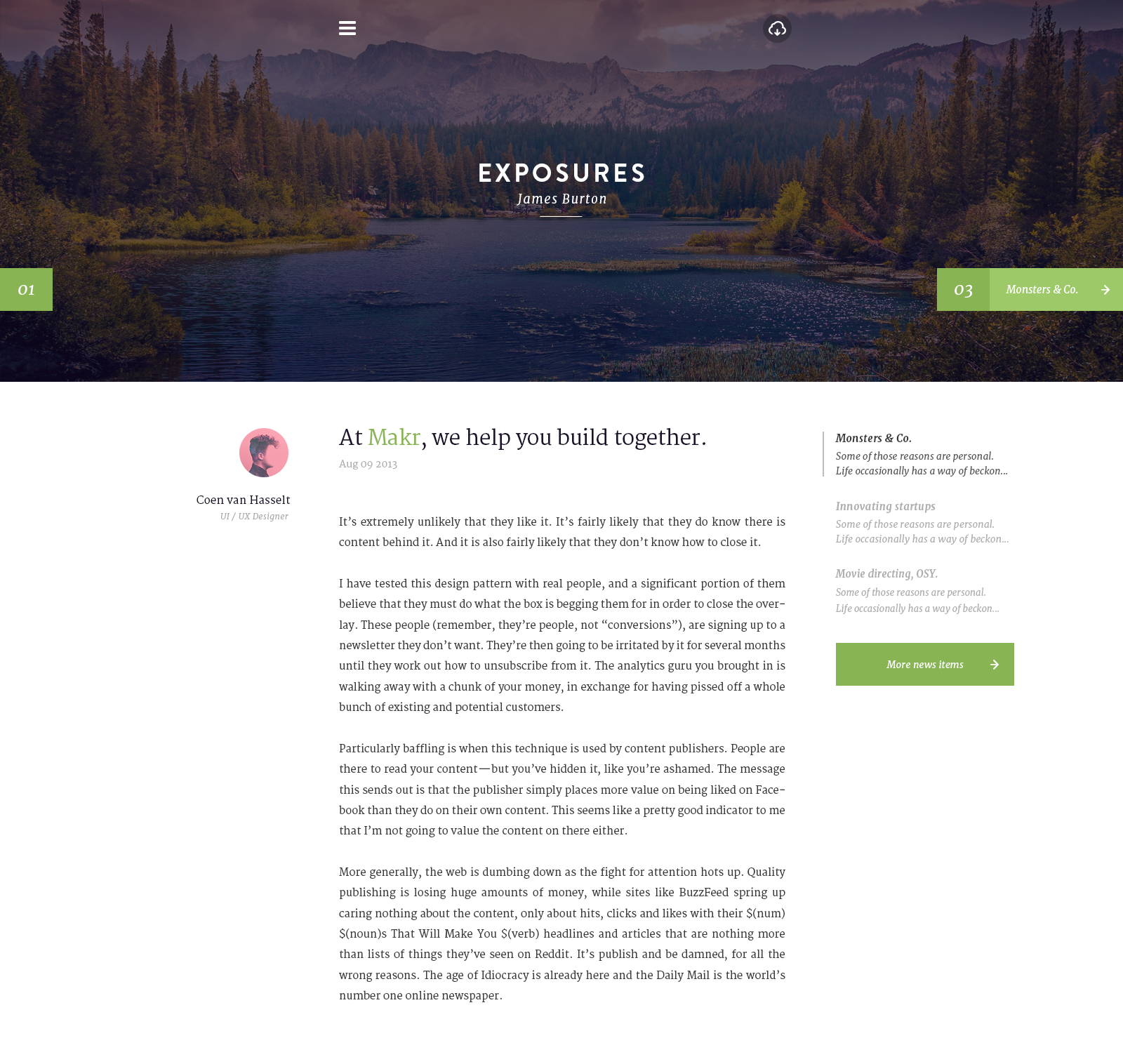This image depicts a webpage displayed on a computer screen. The top third of the page showcases a captivating landscape photograph, featuring snow-capped mountains in the background. In the midground, a serene river is flanked by dense pine forests on both sides, interspersed with smaller shrubs along the riverbank. A gentle shadow casts a tranquil aura over the scene.

Prominently positioned in the center of the image is the word "EXPOSURES" in bold, white, capital letters. Directly beneath it, in smaller lowercase font, is the name "James Burton," both elements underlined by a thin white line.

On the left side of the image, a navigation pane is visible, while on the right, there is a cloud icon with a download symbol. At the bottom left corner, a green box with the number "01" in white font can be seen. Conversely, on the bottom right, another green box contains the number "03," accompanied by the text "MONSTERS AND CO." and a right-facing arrow.

Below the main image, the webpage continues with a body of text. The title at the top reads, "At MAKR we help you build together," with "MAKR" highlighted in green. Beneath this title is a date: August 9th, 2013. To the left, there is an image of a person against a pink background, although the face is not visible. The caption for this image reads, "KONE VAN HASSELT, UI/UX Designer."

On the right side of this section, another segment labeled "MONSTERS AND CO." contains text that begins, "Some of those reasons are personal, life occasionally has a way of beckon..." Below this, the text "Innovating startups" and "movie direction OSY" can be found. Finally, a green box with the words "MORE NEWS ITEM" and a right-facing arrow concludes this section.

Overall, the webpage is rich with visual and textual elements, organized to create a visually appealing and informative layout.